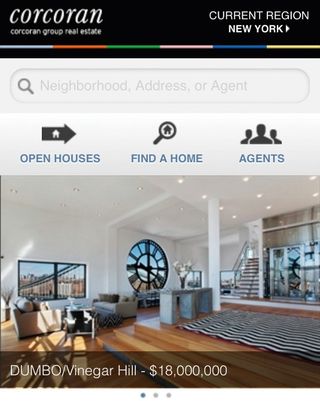This image appears to be a cropped screenshot of a real estate webpage from Corcoran Group Real Estate. At the top, a black bar with white text prominently displays the name "Corcoran, Corcoran Group Real Estate." In the top right corner, it indicates the current region as "New York." Just below this section, a multicolored bar is visible, acting possibly as a navigation or selection tool. Beneath the multicolored bar is a gray search field containing light gray text that reads "neighborhood, address, or agent," accompanied by a magnifying glass icon to the left.

The subsequent gray rectangle hosts three distinct icons and corresponding labels in blue: an arrow with a house labeled "Open Houses," a magnifying glass with a house labeled "Find a Home," and silhouettes of three individuals labeled "Agents."

Directly below these icons, there is a photograph showcasing the interior of a spacious living room. The room features an elevated section, a large window, a clock-shaped window, and a couch on hardwood flooring. At the bottom of the image, a translucent black rectangle with white text provides specific details about the property: "Dumbo/Vinegar Hill - $18 million."